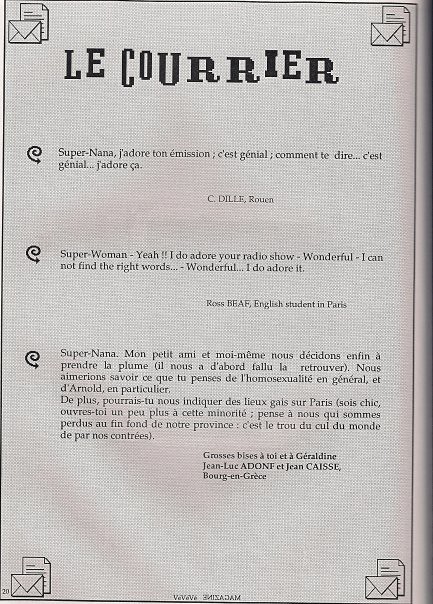The image depicts what appears to be a page from a booklet or a newspaper titled "Le Courrier." The page has a white background with a slightly grayish hue and a black border on the right side, with scattered reddish faded patches throughout. At the top, the heading "Le Courrier" is prominently displayed in dark black font. Each of the four corners features an icon of an envelope with a page behind it.

The content consists of three testimonials or quotes, two in French and one in English, seemingly related to a radio show. The first quote is from "C-D-I-L-L-E, Rouen" and is in French, beginning with "Super Nana." The second, from "Ross B-E-A-F, English student in Paris," is in English: "Superwoman, yeah, I do adore your radio show. Wonderful. I cannot find the right words. Wonderful. I do adore it." The third quote, also starting with "Super Nana," is written in French and attributed to "Jean-Luc A-D-O-N-F."

Overall, the page seems to be a collection of international testimonials or reviews about a popular radio show, visually distinguished by the envelope icons and mixed-language excerpts.